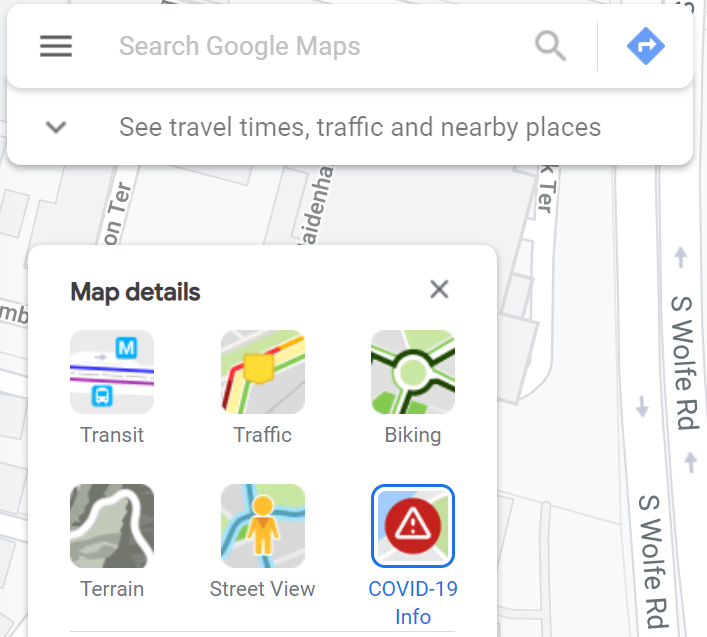The image displays a smartphone screen with the Google Maps app open. At the top-left corner, there is a hamburger menu icon, followed by a magnifying glass icon for search, a right-turning arrow, and a blue diamond road sign. Just beneath these icons, there is a drop-down option allowing users to view travel times and traffic in nearby locations.

In the background, the detailed Google Maps interface is visible. An overlay panel labeled "Map details" is overlaid on the map, featuring a legend or key. It indicates various elements available for viewing:

- Roads with a bus icon and an "M" symbolizing metro or transit options.
- A "Transit" label for public transportation options.
- Traffic conditions displayed in colors: yellow, red, orange, and green.
- Biking routes marked with green icons.
- Roads shown in black, white, and gray on a terrain field.
- A person walking icon, likely representing pedestrian paths.
- A "Street View" icon for a street-level view.

Additionally, there is a blue-bordered area with blue text reading "COVID-19 info," indicated by an exclamation mark inside a white triangle within a red circle. 

Both the overlay panel and the header bar, which includes the search function, have a drop shadow giving them a distinct appearance against the monochrome base map displayed underneath. However, the actual map does not show any of the items detailed in the map legend.